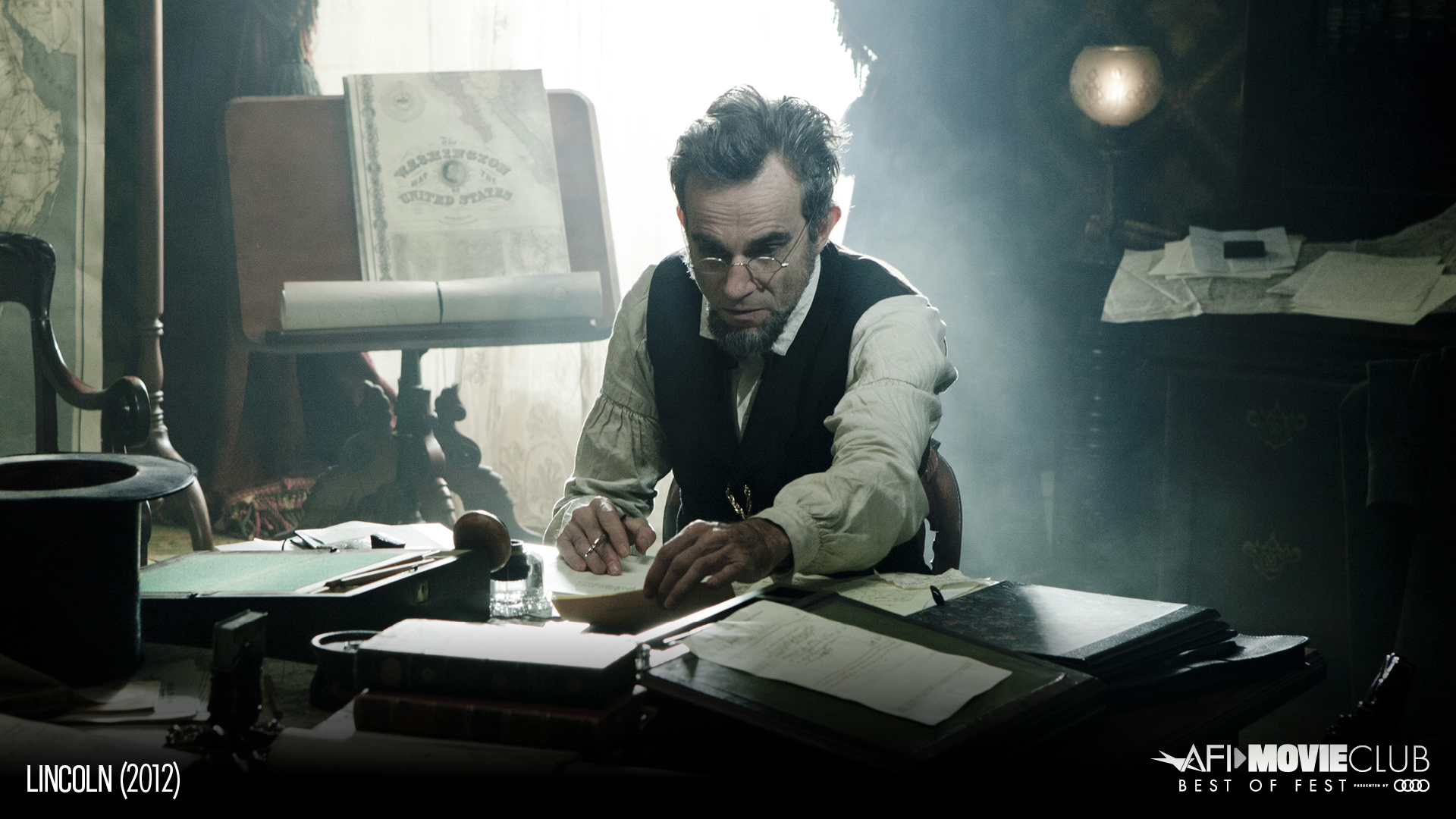The poster for the 2012 movie "Lincoln" prominently features Daniel Day-Lewis as Abraham Lincoln, seated at a cluttered desk. He is meticulously studying and writing on papers spread out before him, a pen in his right hand. His iconic tall hat rests on the desk's left edge. Lincoln's characteristic glasses sit on his face, and he is dressed in a white ruffled dress shirt and a black vest, complete with his iconic goatee. The scene is set in a softly lit room, with a lantern over his left shoulder and an open window behind him, allowing light to stream in. To the right, behind him, a stand holds a large document and a rolled-up parchment amid numerous additional papers. At the bottom left of the poster, the title "LINCOLN (2012)" is displayed in bold white capital letters. The bottom right corner features the AFI Movie Club logo and the "Best of Fest" accolade, with the Audi logo indicating a likely sponsorship. The image conveys the intense dedication and intellectual fervor of Lincoln, as portrayed in this critically acclaimed biographical film.